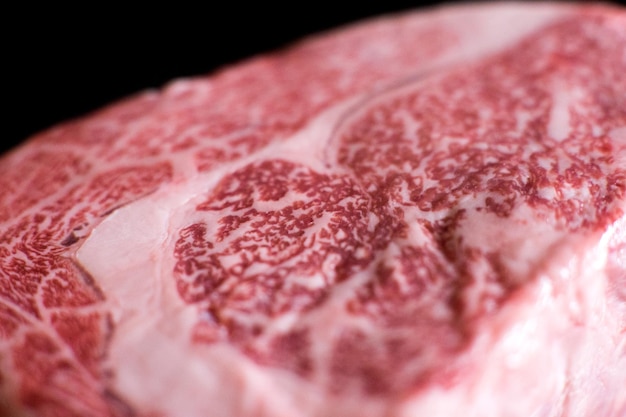This image is a close-up shot of a raw piece of beef, most likely a steak or roast. The background is predominantly black, providing a stark contrast that highlights the details of the meat. The raw beef is characterized by a range of reddish to pinkish hues, showing varying shades from lighter pink to darker red. The left edge of the meat features a substantial, curved section of fatty tissue, which wraps around part of the darker meat. Marbling is visible throughout, with a large collection of fat in the middle and smaller veins of fat dispersed across the meat. The right edge of the image shows the side of the beef, slightly out of focus but illuminated, adding depth to the close-up shot. The overall composition draws the viewer's eye from the lower left to the upper right, emphasizing the texture and richness of the raw meat.